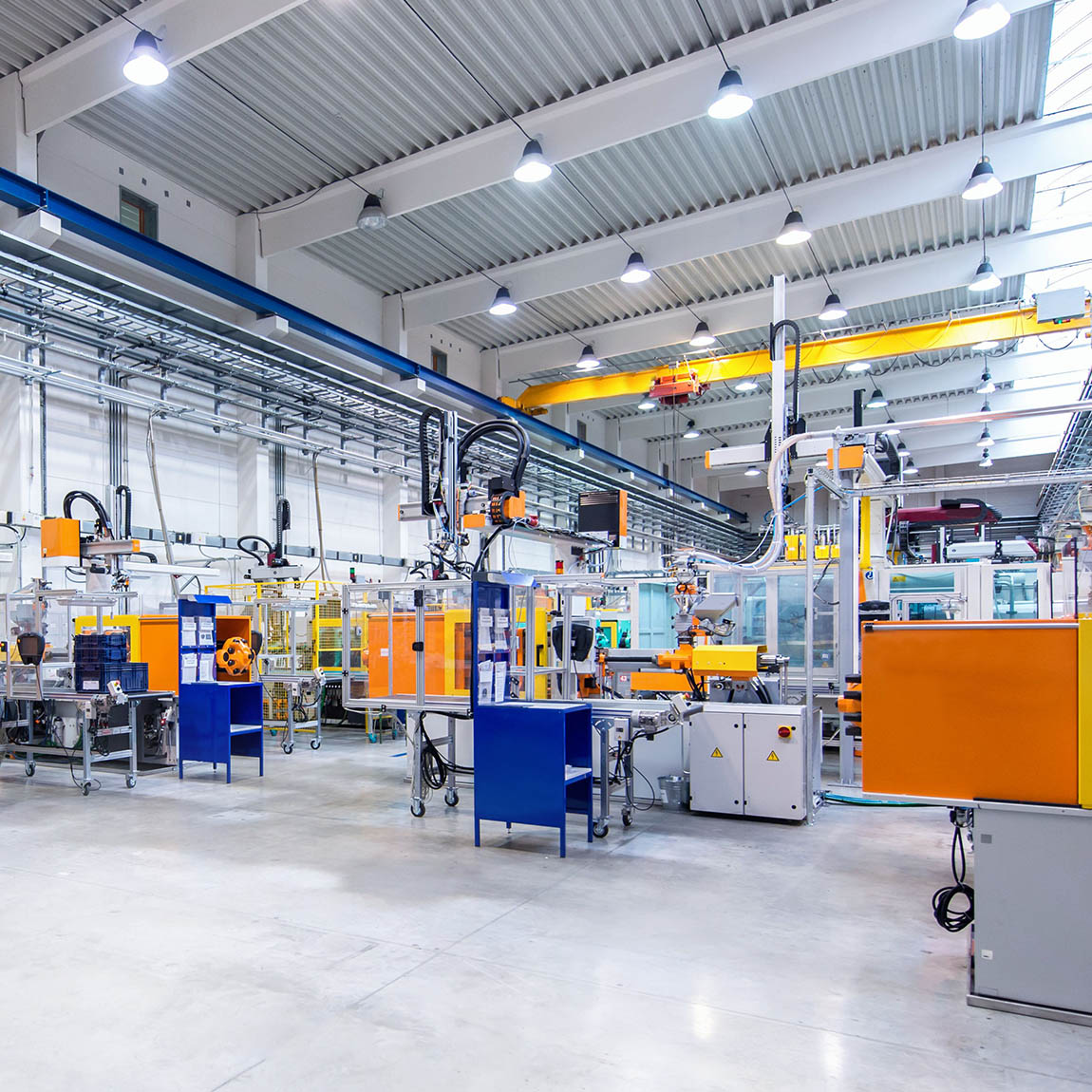The image depicts an intricately organized, brightly lit industrial area, resembling a factory floor or laboratory. The interior, dominated by sheet metal with a whitish or light gray hue, gives a sleek and modern feel. Overhead, numerous LED lights illuminate the area intensely, contributing to the crisp visibility in the photo. The floor, made of light gray concrete, appears spotless, enhancing the overall impression of cleanliness and newness.

Various workstations and cubicle-like areas pepper the environment, featuring striking colors like deep royal blue, school bus yellow, and Home Depot orange, which contrast vividly against the monochromatic backdrop. These areas house neatly organized equipment, tables, and tools. Among the fixtures, hoses and wires snake through the space, suggesting industrial assembly or laboratory processes.

Prominent steel girders, painted in vibrant yellow and blue, span the width and length of the room, respectively, adding structural emphasis. Additionally, there's a visible overhead system showcasing HVAC and plumbing elements. The absence of people in the image suggests it might have been taken before operations commenced or during a downtime, leaving the purpose of the facility ambiguous, although the impeccable arrangement and the sophisticated infrastructure hint at advanced manufacturing or laboratory activities.